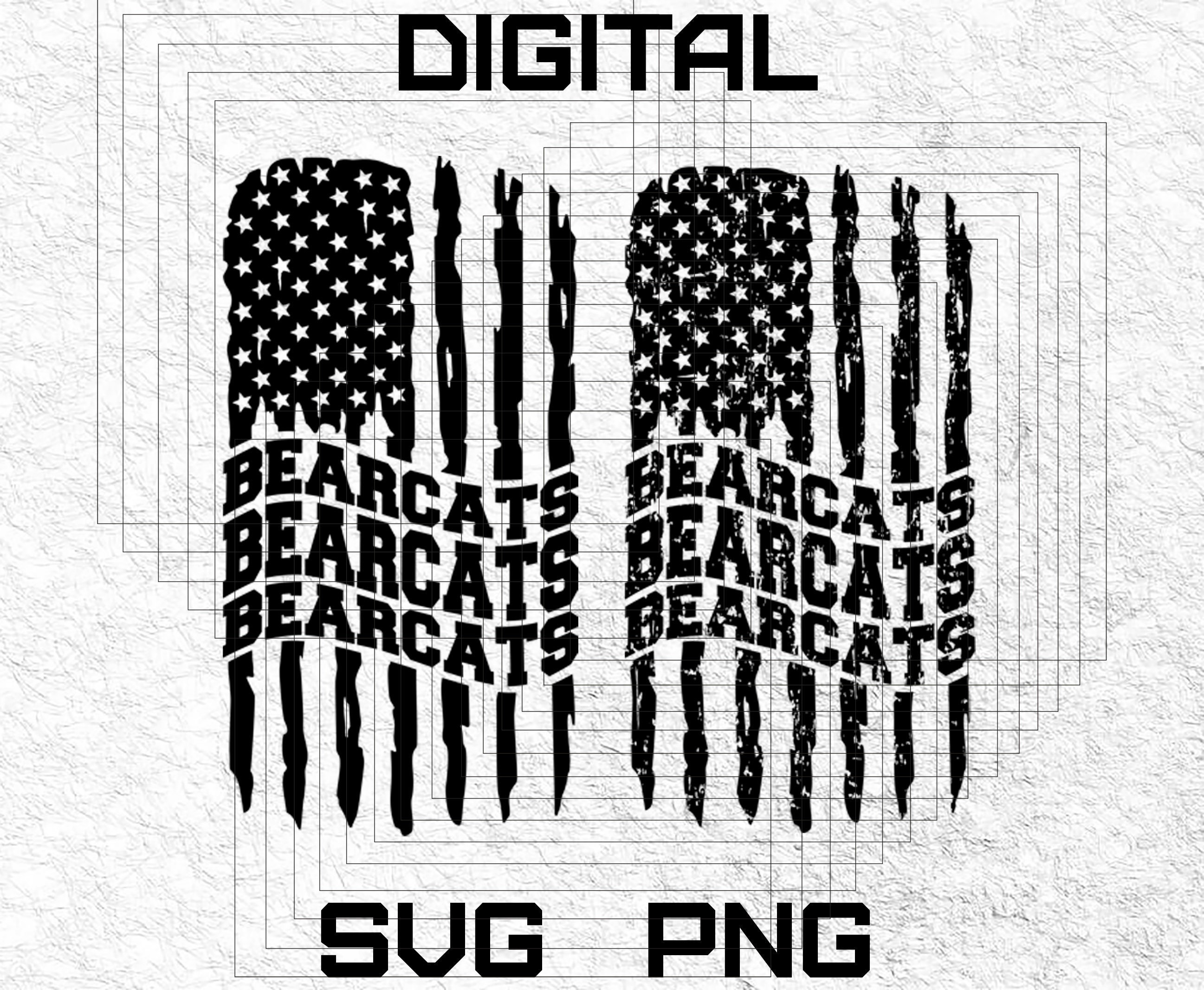This detailed black and white drawing features a textured white background that resembles stucco or a popcorn wall with gray striations. At the top of the image, the word "digital" is boldly written in large black letters. Centrally, there are two distressed American flag motifs positioned side by side, each appearing as though clawed or tattered. These flags have stars in the upper left sections and wavy stripes extending downward. Between the two flags, the word "Bearcats" is repeated three times in a row: "Bearcats, Bearcats, Bearcats." At the very bottom of the image, the large black words "SVG" and "PNG" are prominently displayed.